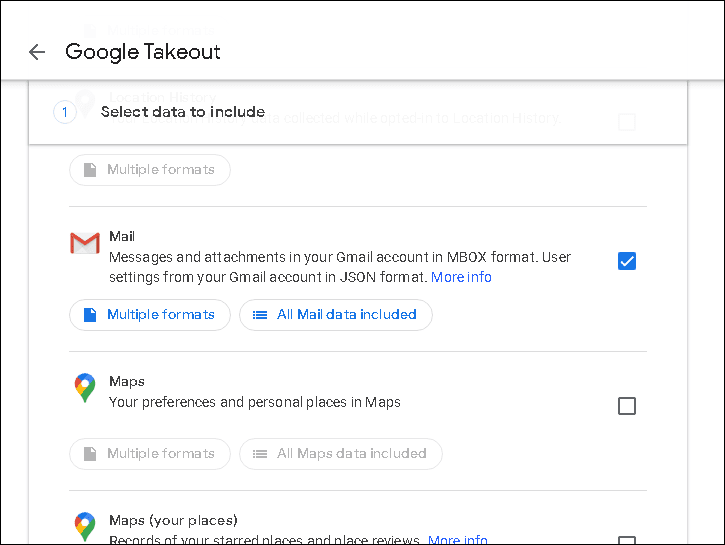The image is a user interface for Google Takeout, designed to guide users through the process of selecting data for export. The rectangular image is approximately 20% wider than it is tall and is bordered by a thin black line against a white background.

In the upper left corner, a back arrow icon is followed by the text "Google Takeout" in black. Below this, the interface is divided into sections by horizontal gray lines.

The first section is marked with a light blue number "1" inside a circle, accompanied by the black text "Select Data to Include." Beneath this, there is a grayed-out button featuring a page icon and the text "Multiple Formats," indicating that this option is currently inactive.

The next section begins with the Google Mail icon and the word "Mail" in black text. Underneath, it describes the types of data to be included: "Messages and Attachments in your Gmail account in mbox format, User Settings from your Gmail account in JSON format." A blue "More Info" link is also present. A checkbox beside the section title is marked with a blue check, indicating that this option has been selected. This section also includes two additional buttons: "Multiple Formats" and "All Mail Data Included."

Following another dividing line, the next section features the Google Maps icon and the label "Maps," with a description below stating: "Your Preferences and Personal Places in Maps."

These elements collectively guide the user in selecting specific Google data to export through the Google Takeout service.